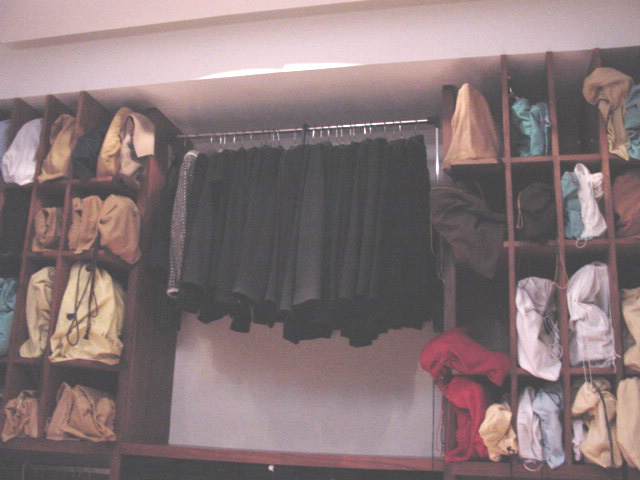The image depicts a well-organized wardrobe closet designed with dark-stained wooden shelving, creating a sophisticated look. The closet features a centrally positioned metal bar, from which an array of black clothing items—likely suit jackets or pants—hang uniformly on silver hangers. On either side of the metal bar, the closet walls are adorned with brown cubic shelves of varying vertical slots, filled with neatly arranged clothing items. The items within these shelves are predominantly in shades of beige, khaki, white, blue, green, and red, resembling a collection of folded clothes or linen bags. The top section of the image shows the white walls and ceiling, highlighting the horizontal rectangular shape of the closet. On the far left, an individual coat or sweater with gray and white tones stands out among the otherwise dark hanging garments. Beneath the hanging clothes, additional brown shelving offers further storage space.